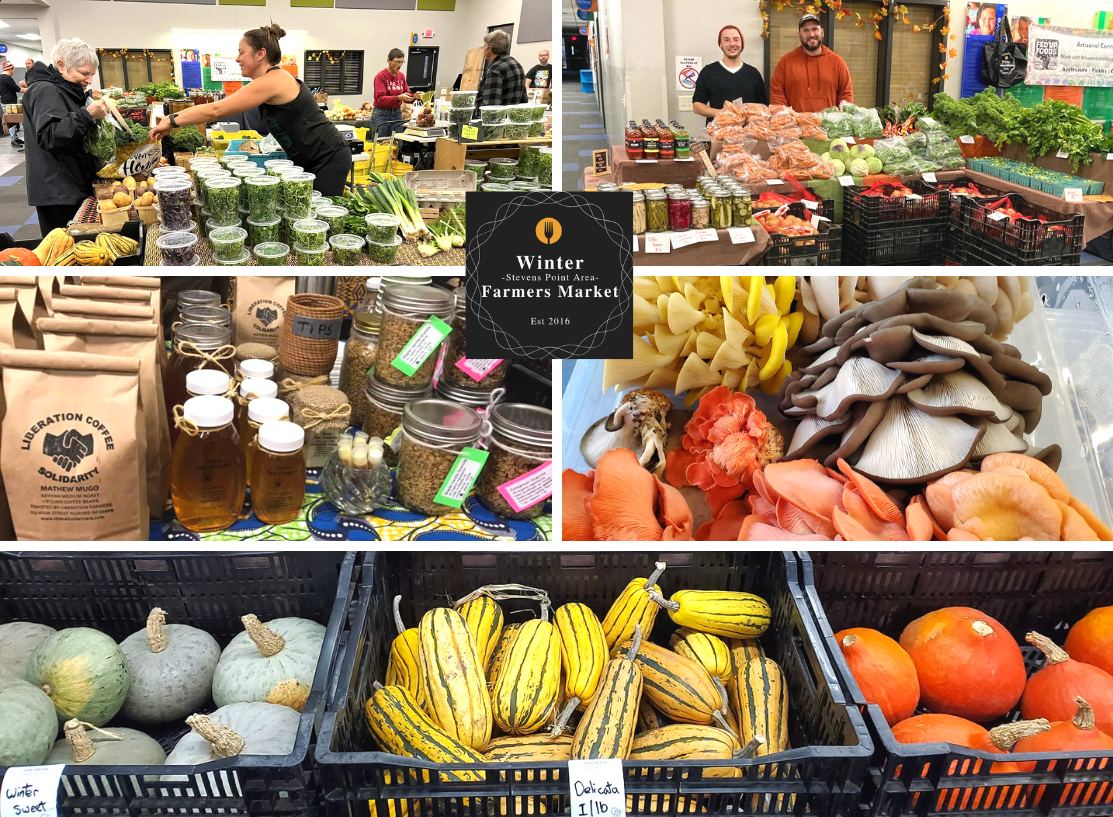The image is a composite advertisement for a Winter Farmers Market, showcasing a vibrant collection of scenes from the market, including both shoppers and an array of fresh produce. The top left photo features a woman with a ponytail in a black tank top, reaching over a counter lined with translucent containers brimming with green leafy vegetables, such as lettuce and celery, alongside squash and zucchini. The adjacent image to the right depicts a man in an orange hoodie and another in a dark-colored shirt, positioned behind tables laden with bags of carrots, whole heads of cabbage, and red netted bags of onions. In the bottom right corner, there are white pumpkins juxtaposed with other vegetables that might resemble upside-down tomatoes. The scene emphasizes a variety of produce, including jars of honey, brown mushrooms, and a range of colorful vegetables—yellow, red, and green. Central to this advertisement, marked prominently with the text "Winter Farmers Market," are the dynamic interactions and transactions between the vendors and customers, all encapsulated in a series of vivid, detailed photographs.